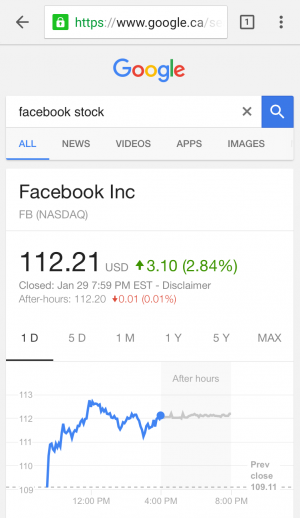Screenshot of a Google search on a smartphone:

The top left corner features a left-pointing arrow, indicating the option to go back. Adjacent to the arrow is the URL bar displaying "https://www.google.ca" followed by a black box with the number "1" inside. To the right of this box is a three-dot icon, suggesting additional options.

Below the URL bar, the iconic Google logo is prominently displayed, followed by another search bar containing the query "Facebook stock." This search bar includes a gray "X" on the right side for clearing the text and a white search icon within a blue box for initiating the search.

Following the search bar, navigation options are listed horizontally: "All," "News," "Videos," "Apps," and "Images."

The main content area features information about Facebook Inc. (FB), listed on NASDAQ. The stock price is shown as $112.21 USD, indicating an increase of $3.10 or 2.84%, with all figures displayed in green. Additionally, the text notes that the market closed on January 29th at 7:59 PM Eastern Standard Time. A disclaimer follows, showing the after-hours price as $112.20, a minimal decrease of $0.01 in red.

Below this section, various time frame options—1D (1 day), 5D (5 days), 1M (1 month), 1Y (1 year), 5Y (5 years), and Max—are available for viewing the stock's performance. The accompanying graph illustrates the stock's fluctuating price with a blue line that trends upward.